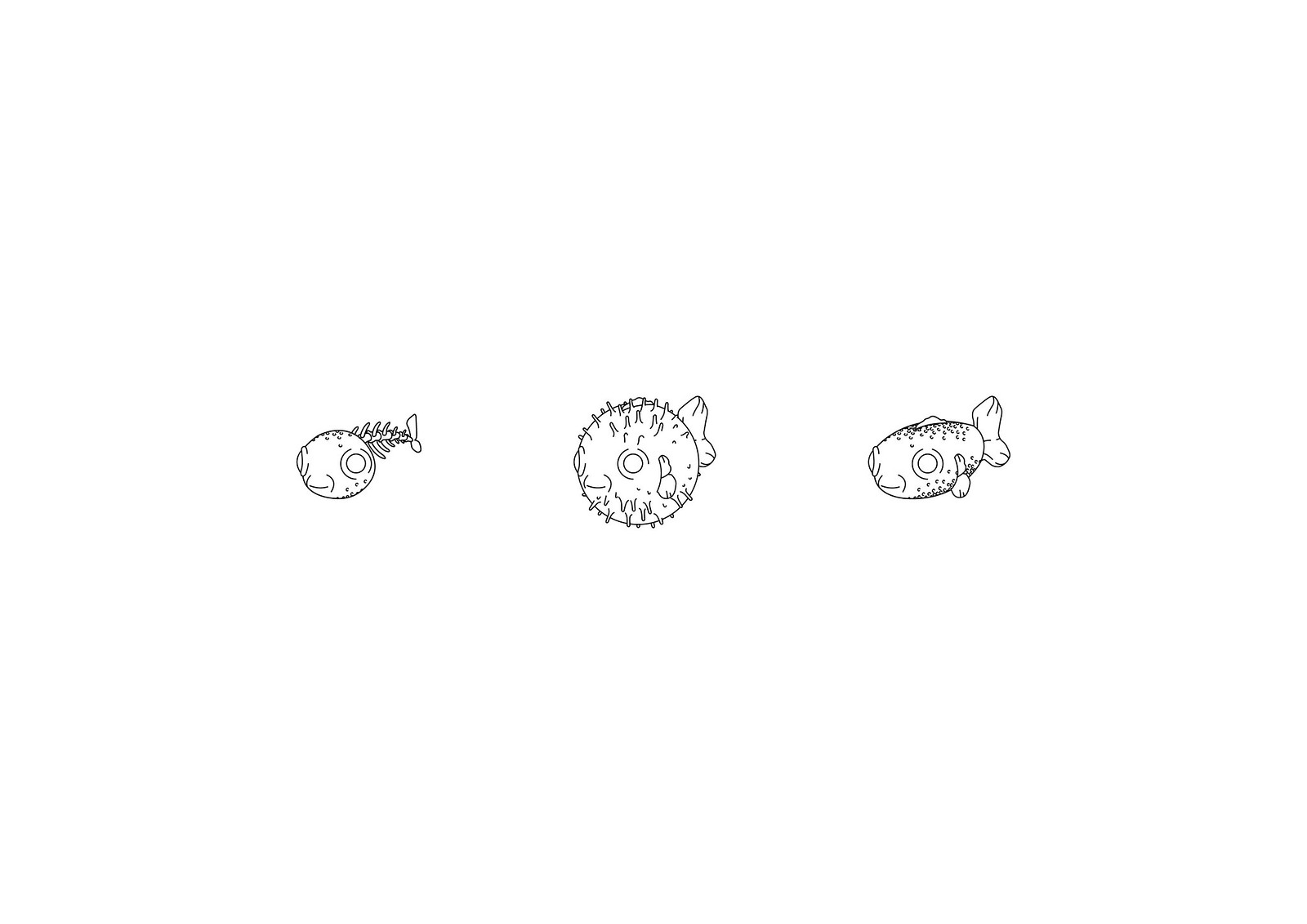This is a detailed black and white sketch on a white background, likely drawn with pen. The image features three drawings of a pufferfish, arranged horizontally and shown in a three-quarter profile with the head to the left and tail to the right. The first drawing on the left depicts the pufferfish with a round head and an exposed spine, resembling a skeletal form where the body appears virtually absent except for the visible rib bones and tail. The middle drawing shows the pufferfish fully inflated, its body transformed into a perfect round shape with noticeable spikes protruding and the fins are positioned at the back. The eyes, which have no pupils, are represented as simple circles. The third drawing on the right shows the pufferfish in its deflated state, appearing as a typical nondescript fish with the same circular eyes and a more oval-shaped body. The spikes are not visible in this depiction, giving it a smoother texture compared to its inflated form. The simplicity and consistency of line work emphasize the transformation of the pufferfish across its different states.